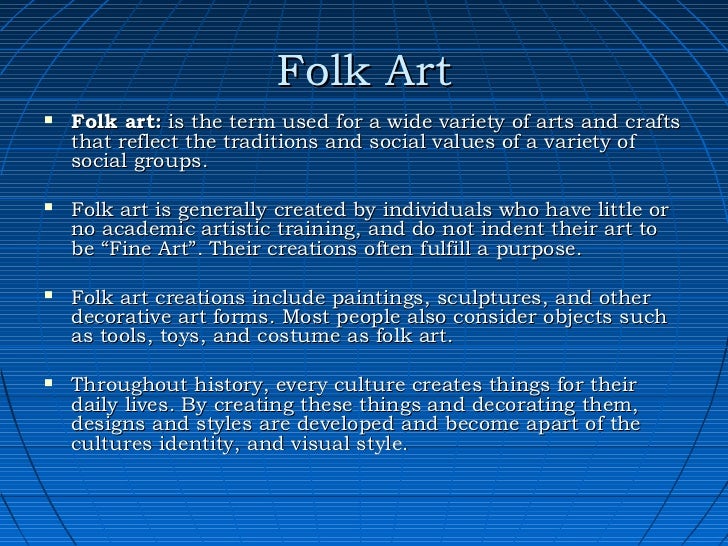The image appears to be a screenshot from a slideshow presentation, featuring a dark blue background interlaced with a lighter blue grid of horizontal and vertical lines, creating a globe-like appearance. At the center, "Folk Art" is prominently displayed in white letters, followed by a series of four bullet points. The first bullet point defines folk art as a term that encompasses a wide range of arts and crafts embodying the traditions and social values of various social groups. The second bullet explains that folk art is typically created by individuals with little or no formal artistic training and is not intended to be classified as fine art; these creations often serve a functional purpose. The third bullet lists examples of folk art, including paintings, sculptures, and other decorative pieces, while also highlighting that objects like tools, toys, and costumes fall under this category. The final bullet point emphasizes that, historically, every culture has crafted items for daily use, and through their creation and decoration, these items have evolved into integral parts of the culture's identity and visual style.